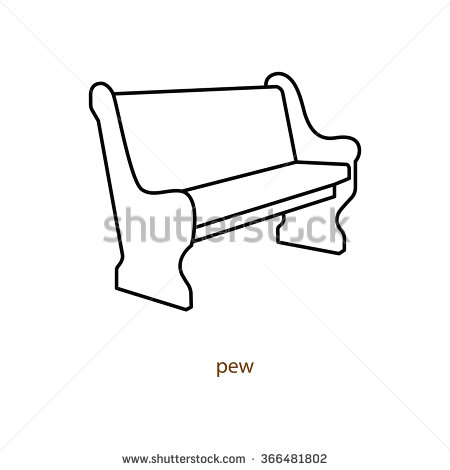The image depicts a simple, black-and-white outline of a church pew, identifiable by its high backrest, sides, and seating area. It features minimalistic details: a small brown lowercase word "pew" beneath the bench illustration. Superimposed over the entire image is a gray, semi-transparent "Shutterstock" watermark, complete with a gray "X" to prevent unauthorized use. At the very bottom of the image, the text "www.shutterstock.com" and the item number "366-481802" are displayed in gray. The background is white, emphasizing the stark simplicity of the drawing and the limited color palette of black, white, gray, and brown.